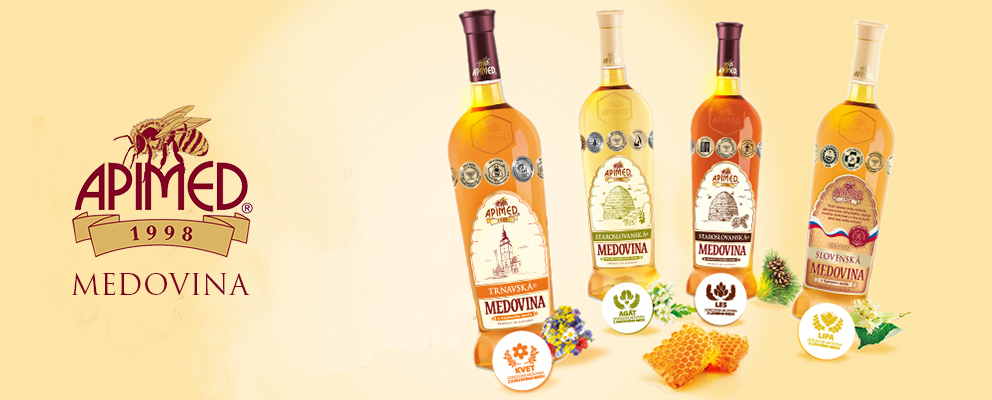The image is a rectangular advertisement for the brand Oppamed Medovina, featuring a light tan background. On the left side, there's a prominent illustration of a bee above the brand name "Oppamed" written in dark red font, followed by a tan banner displaying "1998," and under it, the word "Medovina." To the right, the advertisement showcases four bottles of Medovina arranged in a gentle curve. The bottles exhibit a gradient of colors from light yellow to rich golden honey to dark amber, indicating different flavors or elements derived from various pollinated flowers. Each bottle is topped with purple and white caps. In front of the bottles, two squares of honeycomb are notably displayed, emphasizing the honey-based nature of the drink. The overall hue of the image has a yellow theme that complements the honey and alcoholic tones.